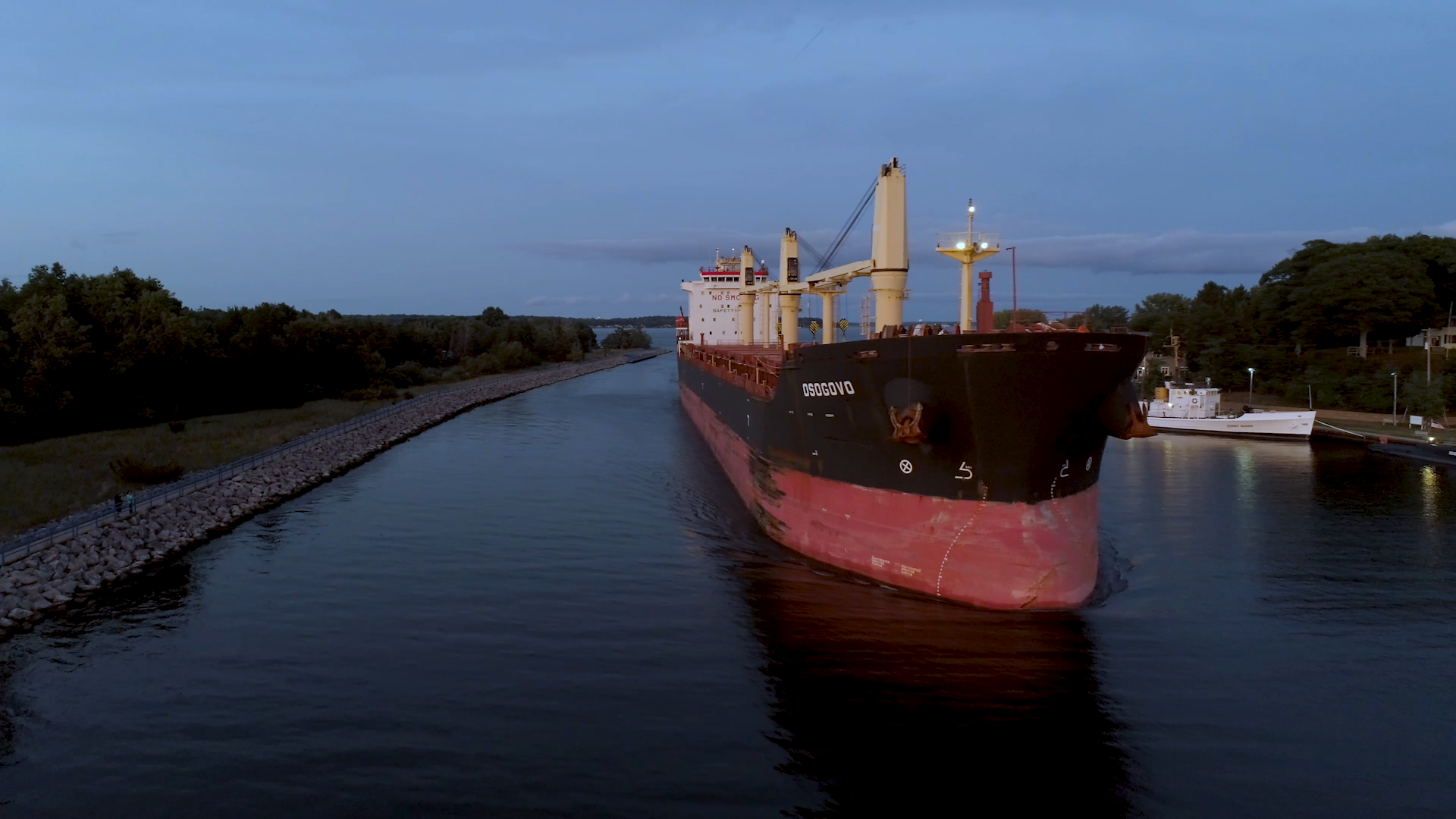The image features a large barge navigating a narrow, calm waterway, possibly a canal or harbor. The forefront of the barge, sporting a weathered black upper section and a faded red base with spots of white showing through, dominates the scene as it moves towards the camera. At the ship’s bow, the letters "O S O G O V O" stand out in white. Above this, a red seating area and cream-colored structures are visible, and towards the rear, a white section bears the cautionary text "NO SMOKING" in red. 

The scene is enveloped in the dim light of dusk, with a dark blue sky occupying the upper third of the image, strewn with scattered, dark clouds. On the left is a grassed bank lined with trees, leading to a tanned stone retaining wall that juts about two to three feet above the water. To the right, amidst more trees, lies a dock where a smaller, white boat is moored. Adjacent to this smaller vessel, a small building peeks into view, indicated by the edge of its roofline. The canal is eerily still, enhancing the tranquil dusk atmosphere, accentuated further by a dual light on the right side of the barge that cuts through the twilight.